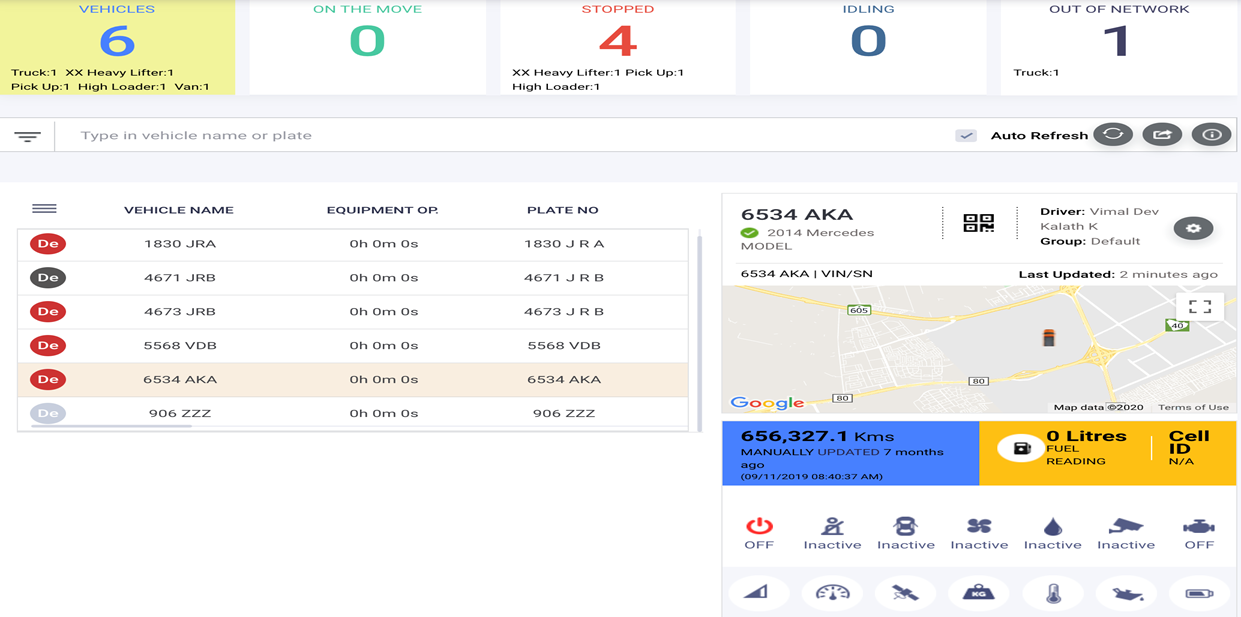The screenshot from a website is partially shown, excluding the top header and footer, making the company or organization's identity unclear. At the top of the visible section, there are five boxes arranged horizontally: four are white, and one on the far left is a very light yellow. Inside the light yellow box, the number '6' and the word 'vehicles' are written in blue. The subsequent boxes, all white, display the following: "On the move" with the letter "O" in green, "Stopped" with the number '4' in red, and "Idling" with the number '0' in blue. The last box on the right corner reads "Out of network" in gray with the number '1'.

Below these boxes, there is a small Google Maps image, with no identifiable labels or names, indicating it is likely depicting a rural area, given the gray background. Further below, two rectangular boxes are present: the left one is blue, and the right one is gold. To the left of these rectangles, there's a chart divided into three columns, although specific details of the chart's content are not visible.